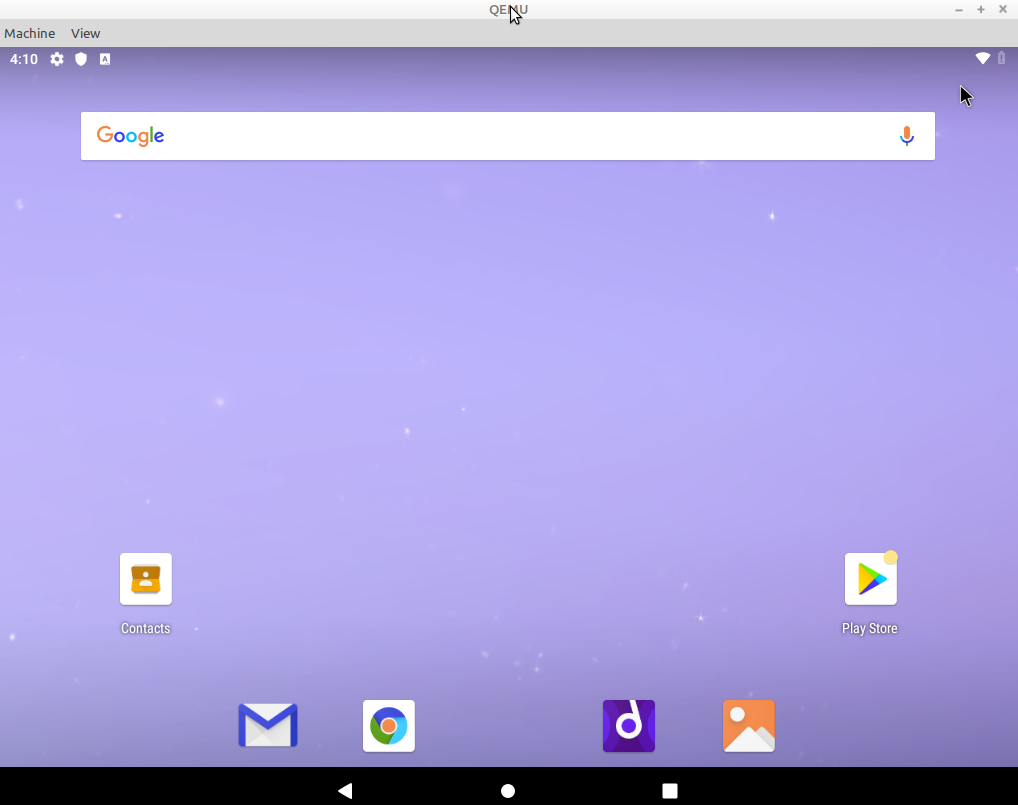The image features a digital interface, likely a screenshot of a phone or tablet home screen. In the upper left-hand corner, the word "machine" appears. Dominating the central area, particularly the middle to top center, is the text "QEMU" in capital letters, partially obscured by a cursor covering the letter "M." 

In the upper right-hand corner, there are three symbols: a minus, a plus, and an X. To the top left of the web page, the time is displayed as 4:10, accompanied by icons for a cog (settings), a shield (security), and a square with the letter "A" (possibly an accessibility or application symbol). 

The upper right corner of the webpage displays a full Wi-Fi signal bar and a battery icon that is not fully charged. Centered at the top of the screen is a Google search bar with the word "Google" on the left and a microphone icon on the right.

The wallpaper displays two apps: the Contacts app in the bottom left corner and the Play Store app in the bottom right. At the bottom center, four bookmarked apps are aligned from left to right: a mailing app, the Google Chrome app, an app marked with the letter "D" or music symbol, and an app depicting a mountain with a sun or circle icon.